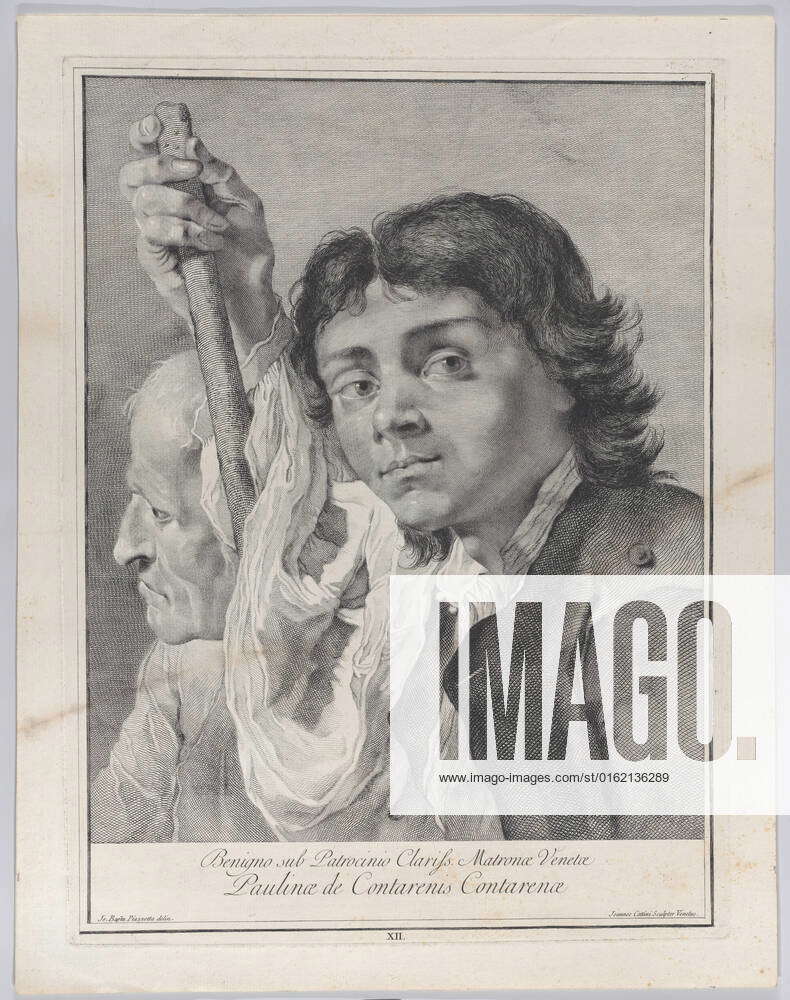This framed poster, encased in a light wood frame with a gray border, presents a close-up digital scan resembling a vintage black-and-white magazine advertisement or portrait. The image, set against a white canvas with a black border, features two figures: a young boy dressed in 18th-century attire with a prominent scarf around his neck and holding a stick (visible only from the mid-chest upward), and an older man, slightly shorter, standing slightly behind. The young boy’s jacket, adorned with buttons, and the older man's white shirt are rendered in a detailed, high-contrast black-and-white style. A cursive text at the bottom of the image reads names such as "Benigno something, Patrocinio, Claris, Matroba, Vene something," followed by "Pauline de Contranes, Contran something." On the right, a white rectangle intrudes into the middle center, featuring the word "IMAGO" in bold, black capital letters, followed by a square period. Below this, a website URL appears: "www.imago-images.com/st/0162136289." The overall aesthetic of the poster combines nostalgic imagery with modern digital enhancement.